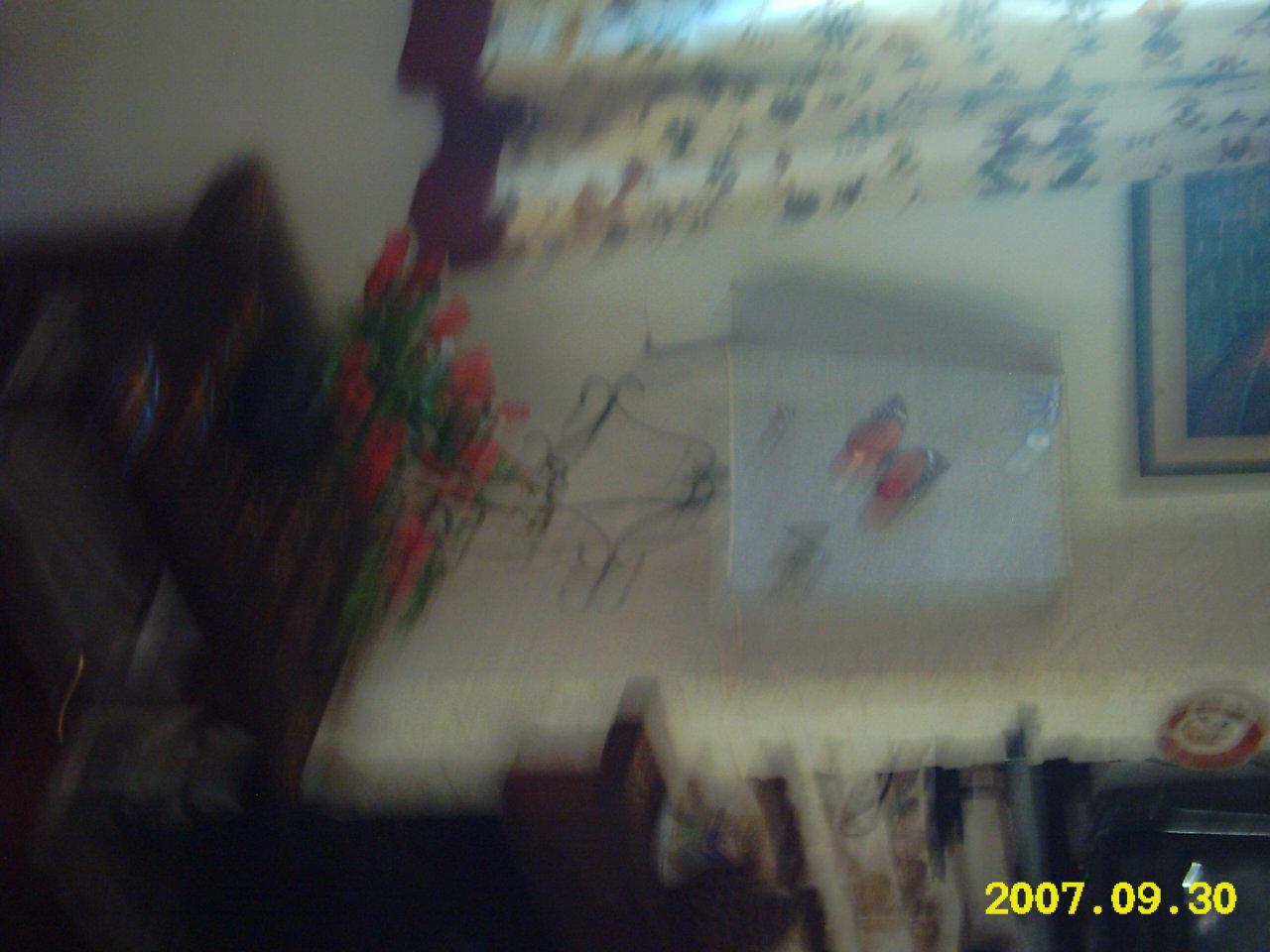This horizontal photograph, taken on September 30th, 2007, captures a somewhat cluttered and blurred interior scene. Central to the composition appears to be a flower vase or a bench adorned with flowers, though the exact nature is unclear. In the very bottom right, there is a hint of yellow coloring, possibly part of the bench or vase. The background is dominated by a white wall, with several indistinct objects including what looks like a red butterfly with black-tipped wings and potentially other insects. Further to the left, there seems to be a black string structure and a bundle of roses.

Above these elements, a white curtain adorned with a blue pattern hangs, featuring triangle shapes and lines, indicative of additional decorative detailing. To the top right of the image, a framed painting with a blue canvas bordered in white within a black frame is visible. The overall image, although heavily blurred and difficult to discern in detail, seems to depict a scene within a domestic setting, marked by a mixture of furniture and decorative elements that create a complex and busy visual impression.